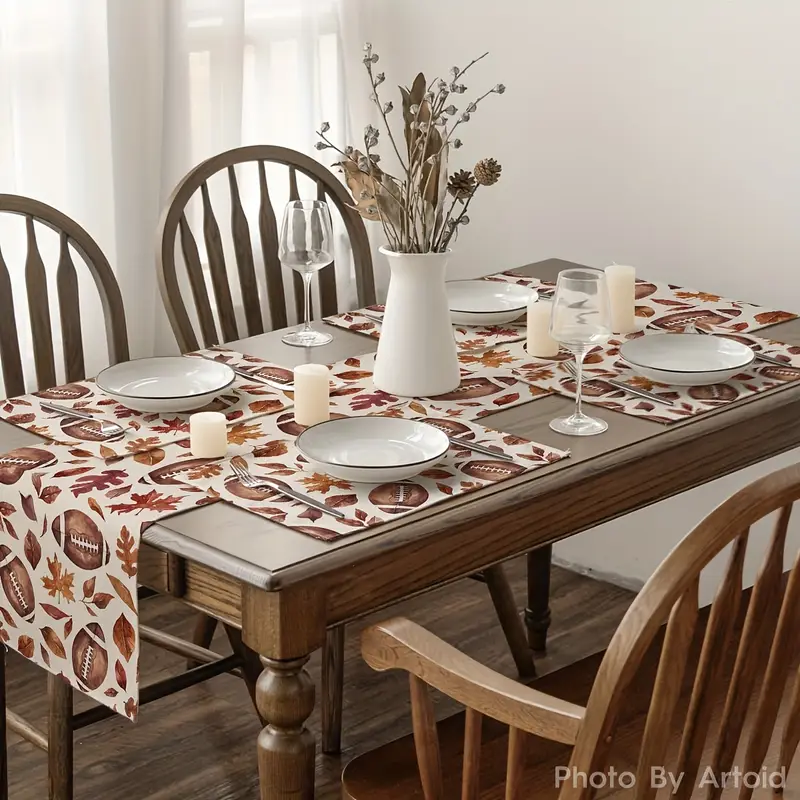This image depicts a cozy small dining room with a wooden, rectangular table set prominently in the center. The room features white walls and white curtains, with sunlight filtering through the window, casting a gentle glow. The table, adorned with fall-themed decor, includes a runner embellished with footballs and autumn leaves in warm fall colors, complemented by matching placemats. Each of the four wooden chairs that surround the table is positioned at a place setting complete with a white bowl featuring a black rim, a fork, a knife, and a wine glass. In the table's center stands a white vase filled with grayish, dry flowers and decorative sticks, giving a rustic touch. Additionally, the arrangement includes four candles – two on each side of the vase. The floor is wooden, enhancing the room's warm, inviting atmosphere. The bottom right corner of the image credits the photographer, noted as "Photo by Artoid."